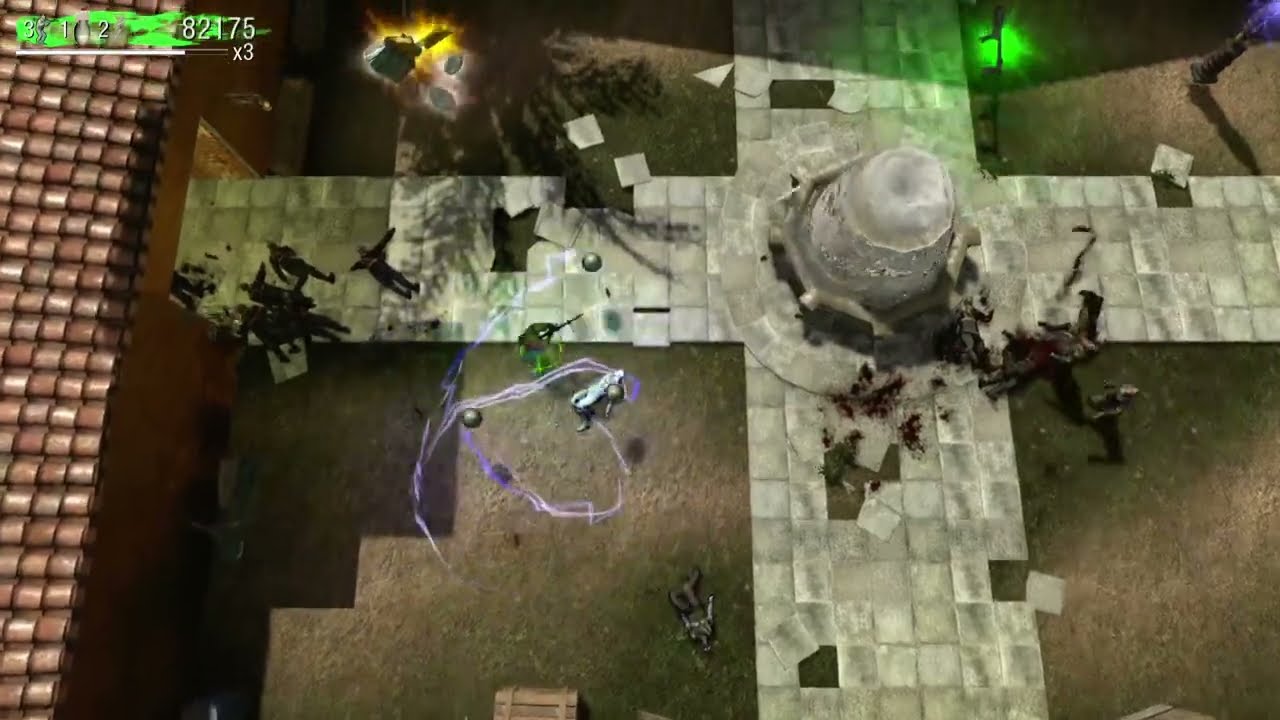The image appears to be a screenshot from a top-down perspective of a video game. Dominating the scene is a white cross-shaped structure made of small white and gray square tiles that intersect, with several of the tiles broken and scattered, as if recently destroyed. This cross intersects a long concrete pathway running horizontally from the open door of a building on the left side of the image. The building is characterized by orangey-brown walls and a roof made of rounded red clay tiles. 

In the middle of the cross-like structure sits a stone fountain on a concrete base. Surrounding the central fountain, several soldiers are positioned, with most lying on the ground, covered in blood. Those still standing appear to be engaged in combat, firing their weapons. There is a patch of grass in the square section between the building and the vertical path, where bodies of soldiers lay sprawled. To the top right, a green shiny light emanates, while to the right, a blue shiny light is visible. 

Additionally, a purple trail swirls around a figure, possibly indicating movement or an active attack. The top left corner of the screen displays game stats in white font with green etching, listing numbers like 82175 and a multiplier of x3. Towards the upper left, a bright, fiery-colored light illuminates the scene, casting a dramatic glow. Overall, the image conveys a chaotic and action-packed moment in a war-torn setting.